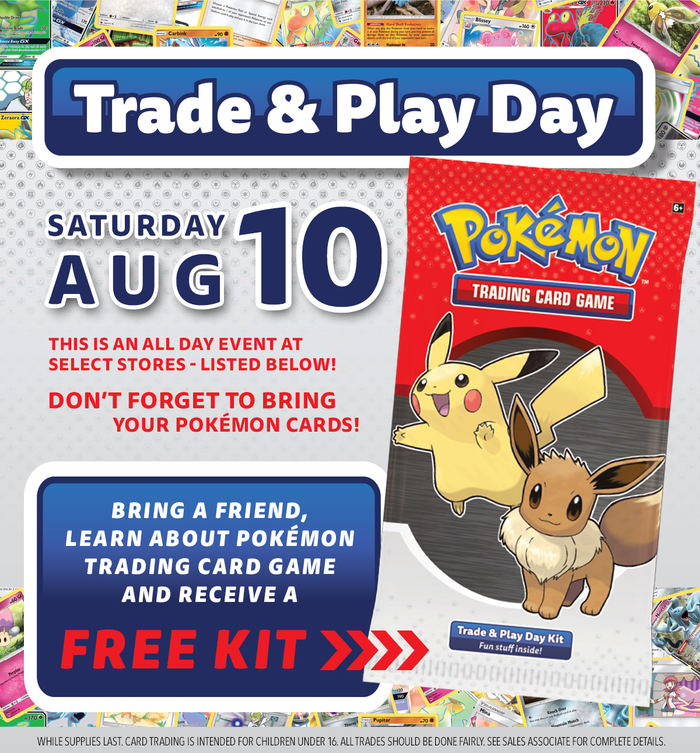This image is an advertisement likely designed for desktop viewing, promoting a "Trade & Play Day" event. The background features a multitude of Pokémon cards, though they are too small to identify without expert knowledge. At the center of the image is a bold blue rectangle with a white highlight, prominently displaying the text "Trade in Play Day."

Below this, in striking blue writing with a white outline, the event date is highlighted: "Saturday, August 10th." Further down, in red writing, the advertisement states: "This is an all-day event at select stores listed below," though no specific stores are visible in the image. The text urges participants not to forget their Pokémon cards.

To the right, an image of a trading card package is shown, featuring the iconic Pokémon logo in yellow with a blue outline, and the words "Trading Card Game" in a red rectangle with a blue outline. The package illustration includes Pikachu, a small yellow creature with orange cheeks, black-tipped ears that stand up, and a yellow lightning bolt-shaped tail. Beside Pikachu is Eevee, a brown, fox-like Pokémon with a large, fluffy collar.

The package promotes a "Trade & Play Day Kit," with a note that it contains "fun stuff inside." At the bottom of the advertisement, a disclaimer reads: "While supplies last. Card trading is intended for children under 16. All trades should be done fairly. See sales associate for complete details."

Overall, this advertisement is for a Pokémon "Trade & Play Day" event, encouraging participants to bring their cards, learn about the trading card game, and receive a free kit.